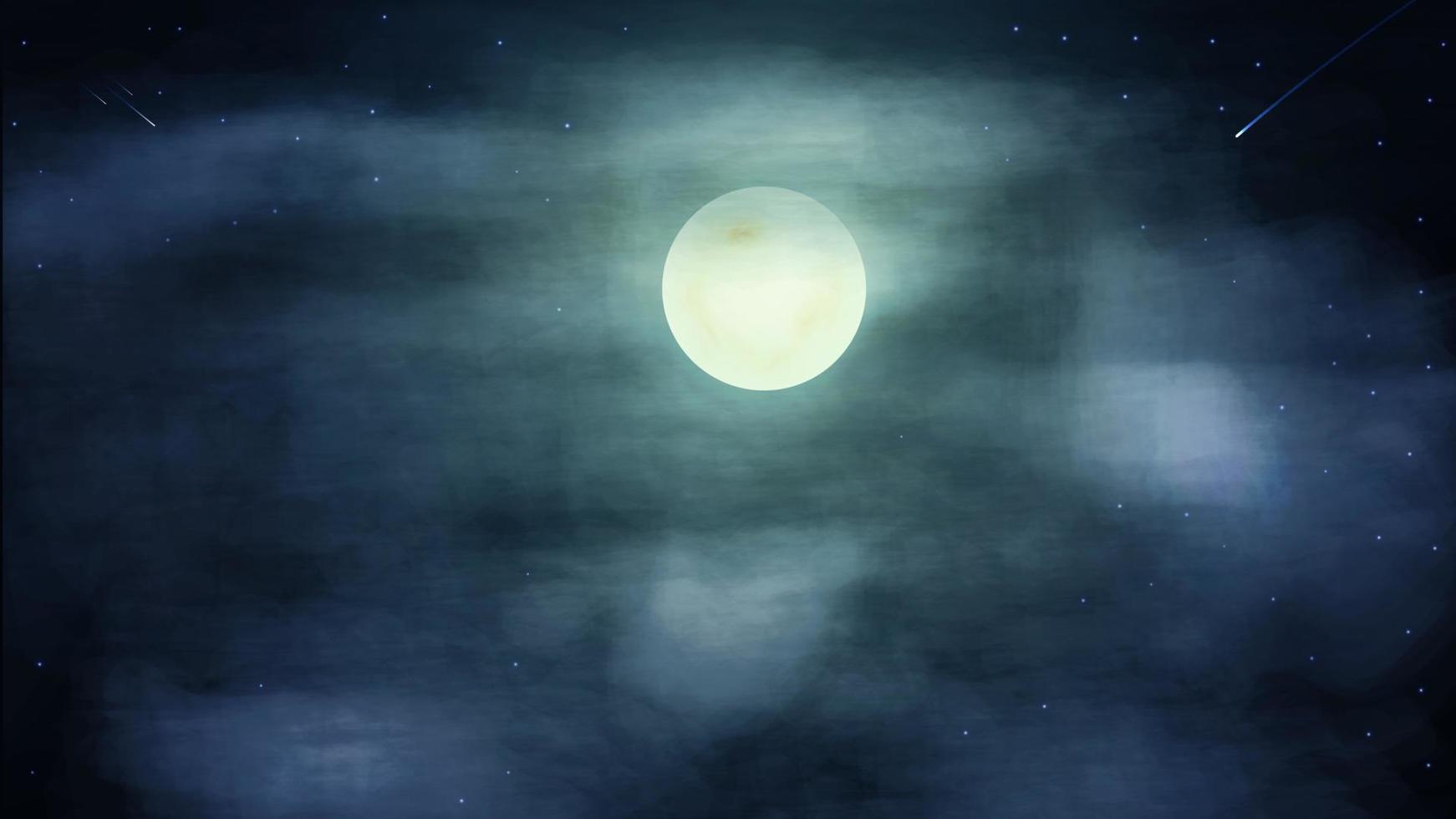This is a digital painting, possibly vector art, which captures the breathtaking beauty of the night sky. Dominating the center, slightly upwards, is a large, glowing full moon in hues of cream white, light yellow, and blue. The moonlight illuminates the sky, creating an ethereal palette of shades, including light green, blue, gray, and even a smoky, semi-transparent glow around the moon. The backdrop is a vast expanse of black and midnight blue, scattered with numerous shining stars, some with a soft, bluish tint. The composition also features shooting stars, a striking one on the top right with a long, comet-like tail, and a few meteors in the top left corner. The meticulous detailing of various colors and celestial elements gives the artwork a serene and magical quality.